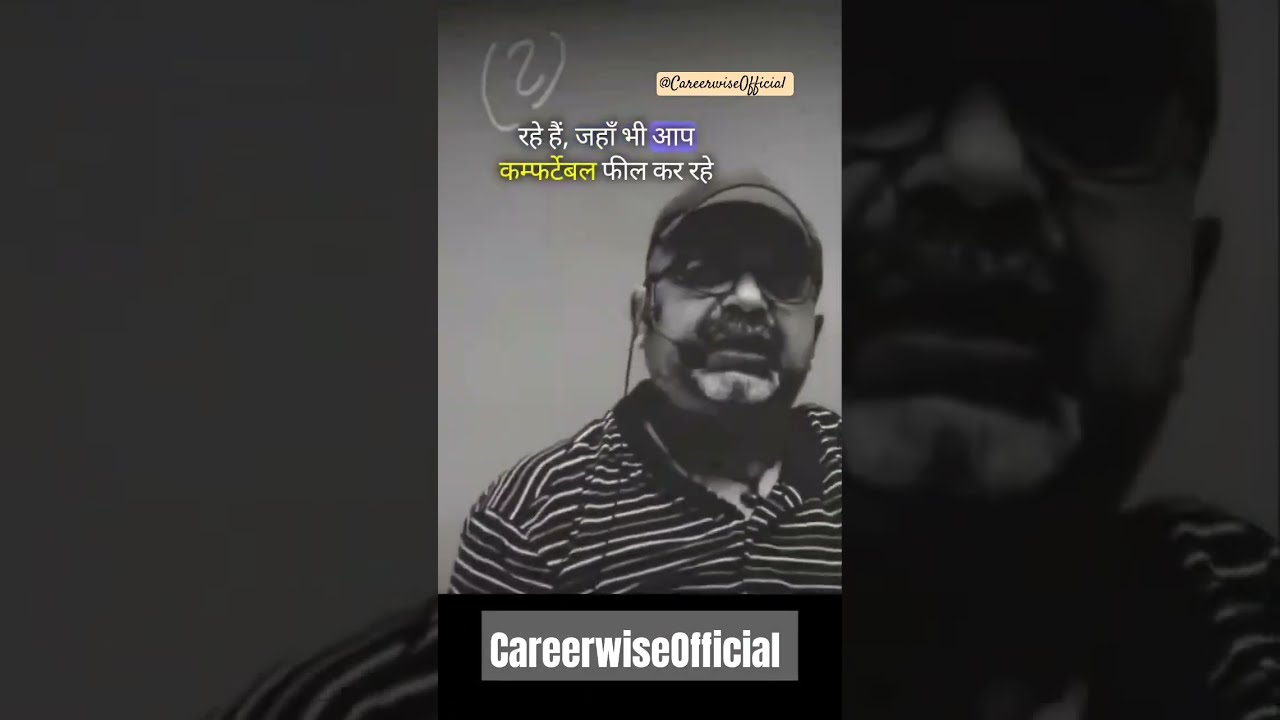This is a detailed grayscale portrait captured in a vertical orientation, inset within an enlarged and darkened portion of the same image stretched to fit a landscape frame. The central image features an older middle-aged South Asian man, slightly overweight, wearing a horizontally striped polo shirt with an open neck and a ball cap. He is sporting glasses, a large mustache, and a salt-and-pepper goatee. The man appears to be speaking into a headset microphone, with the wire visibly hanging down from his ear.

At the top of this central photograph, there is a gray circle containing the hand-drawn numeral "2" flanked by parentheses. Below this, there are two lines of Arabic script; the first line has its last word highlighted in blue, and the second line starts with a word written in yellow. 

To the top right corner of the image, there is a small inset box with a cream background, displaying the text "@CurrywiseOfficial" in a script font. At the bottom of the image, across a black and gray bar, there is the handle "CareerWiseOfficial" written in white font.

The zoomed-in background frames the central image in such a way that on the left side, only part of the man's shirt and the wall behind him are visible, while on the right side, his face minus the left ear, shoulder, and a bit of the background wall are discernible. This image, likely a still from a video or live session, possibly captures the man giving career advice.